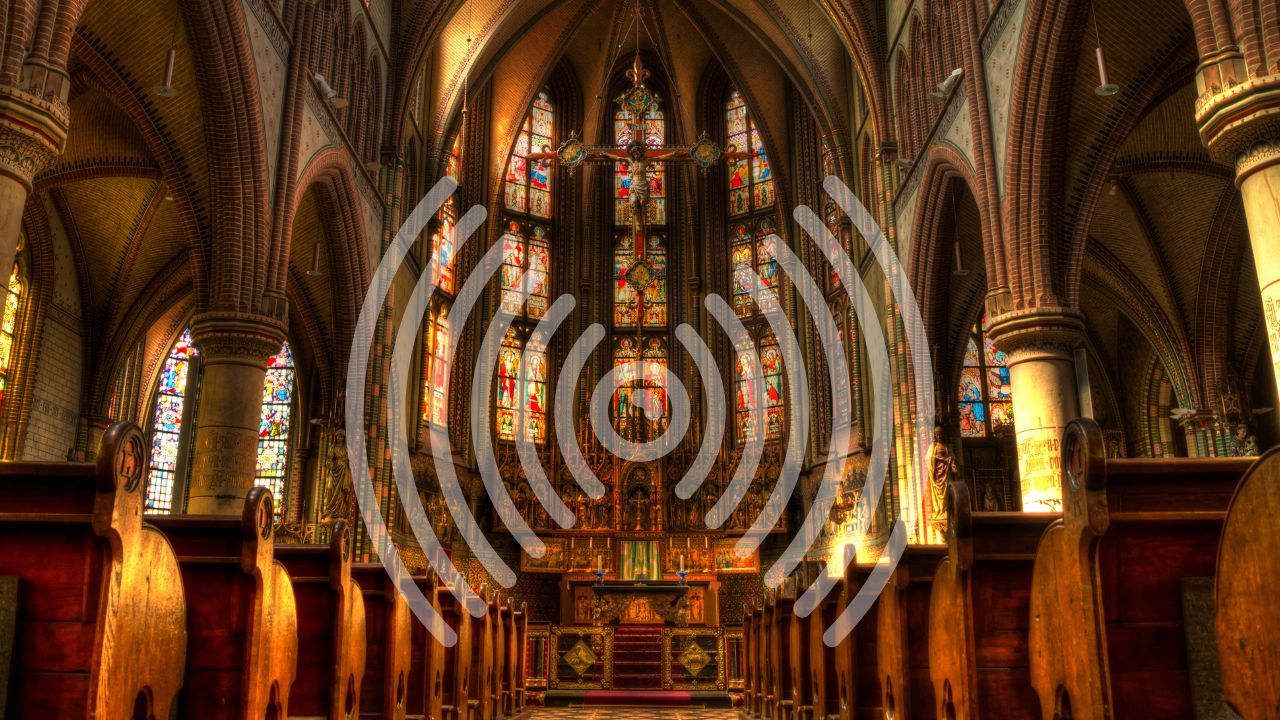This image is a highly detailed, photoshopped depiction of a large AI or CGI church, capturing the essence of an indoor cathedral with a vaulted ceiling. The center hall, adorned with long rows of pews, draws your eye towards the altar or pulpit at the front. Warm autumnal colors—reds, browns, golds, and yellows—illuminate the scene, giving the impression of sunlight pouring through stained glass windows, which are nestled within tall, narrow arches along the sides and at the front of the church. A large, prominent cross hangs from the ceiling, surrounded by ornate archways and additional crosses, signifying the sacred nature of the setting. Overlaid across the center of the image is a semi-transparent watermark resembling radiating semicircles or soundwaves, which adds a modern, technological twist to the otherwise traditional scene. The overlay radiates towards the right or left, subtly altering the visual flow of the image without obstructing the view of the church's richly detailed interior.